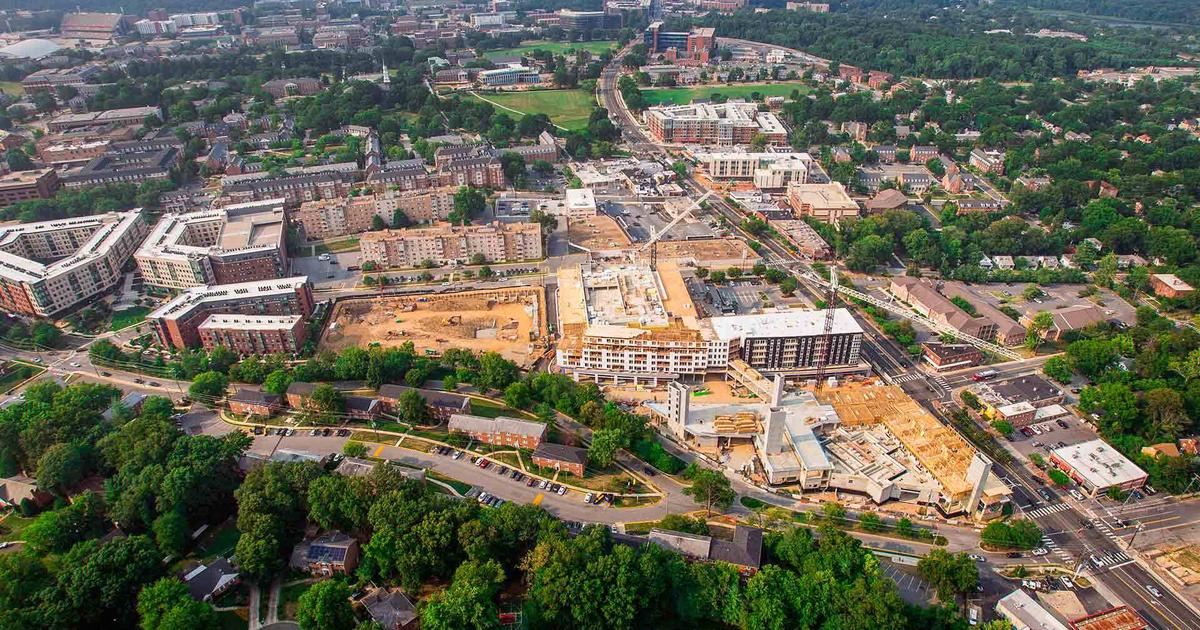This overhead aerial photograph captures a large construction site, potentially for a residential or industrial complex, situated within a city. The image includes a central construction zone characterized by a mixture of completed and in-progress apartment buildings, predominantly red brick with white roofs. Cranes are visibly stationed on some of these six to seven-story structures, with some buildings nearing completion while others are still amidst construction, revealing an expanse of brown dirt and construction materials.

To the lower right of the image, a prominent road runs diagonally, extending towards the center background where it branches off to the left. This thoroughfare is flanked by several clusters of red brick apartment buildings, each separated by rows of green trees, walkways, and parking areas. The upper part of the image showcases more residential buildings and a dense spread of trees lining the roads and freeways, offering a picturesque contrast to the bustling construction activity below.

The detailed layout of the site reveals a triangular section in the center of the image with fewer trees compared to the surrounding areas, emphasizing the planned future expansion. The overall composition highlights the blend of urban development and greenery strategically interspersed throughout the cityscape.